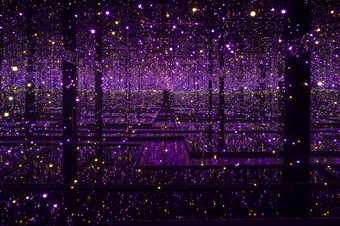This artwork is a dark, purple-hued impressionist painting with an ombre effect that fades to black at the top and bottom. The central focus appears to be a platform or dock extending over water, anchored by high posts that recede into the distance. The scene is enveloped in a mystical atmosphere, with tiny points of light—yellow, white, and light purple—scattered throughout, resembling fairy lights or stars. These lights create a whimsical overlay across the entire image, enhancing its ethereal and fantastical quality. The horizon in the middle emits a purple glow, which subtly illuminates the pathway, adding to the painting's dreamy and enigmatic vibe. Overall, the artwork is dark and fantastical, with a blend of blurred details and vibrant, twinkling lights that evoke a sense of wonder and mystery.